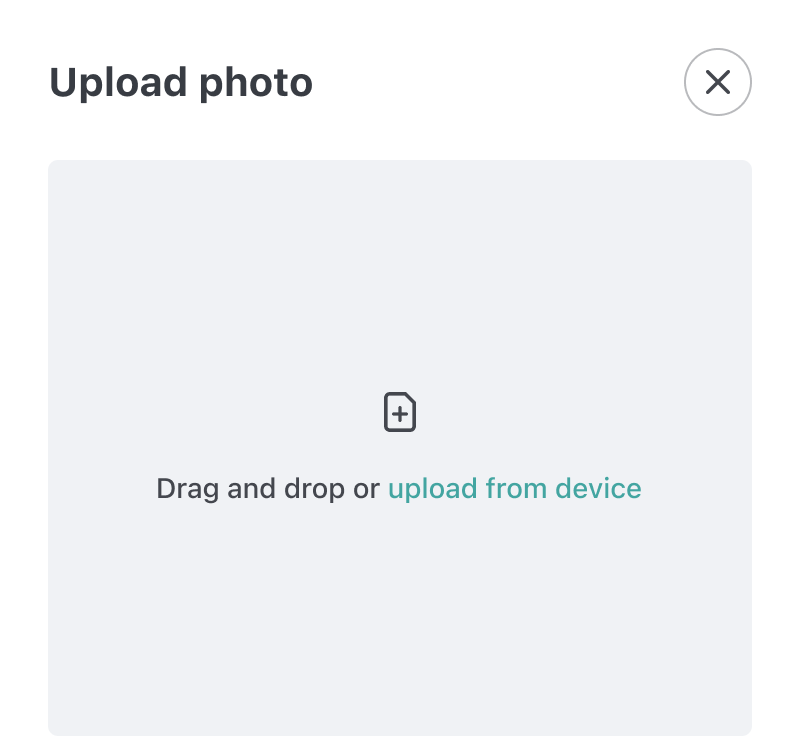Screenshot depicting a file upload interface. At the top, in prominent, bold black font, the heading reads "Upload Photo." Below the heading, there is a medium-sized, circular gray icon with a gray 'X' inside it. Further down, centrally positioned, is a large, clearly defined gray square box. Within this box, there is a dark gray paper icon featuring a plus sign. The box contains text that instructs the user to "drag and drop or upload from device." The phrase "drag and drop or" is rendered in dark gray or black, while "upload from device" is highlighted in teal. The overall image quality is excellent with no signs of pixelation or blurring. The fonts are large, bold, and user-friendly, ensuring clarity. The interface design is clean and minimalistic with no additional images or text to mention. The colors are vivid and distinct, maintaining clear visual separation without any bleeding. The screenshot effectively communicates its intended purpose in a well-organized layout.